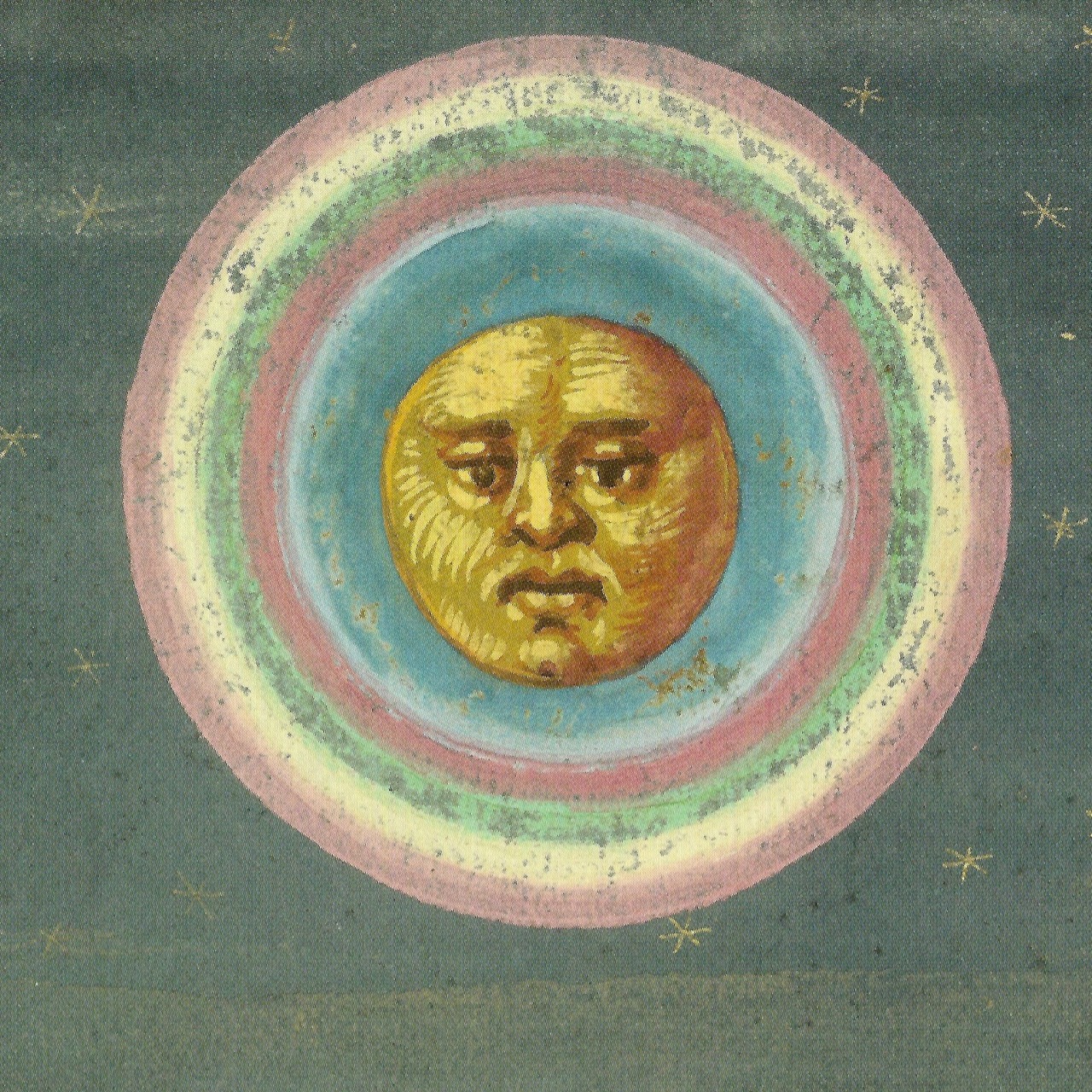This illustration, likely from a children's book, features a square-shaped, whimsical depiction of a celestial body — possibly the sun or moon — against a grainy, grayish-blue background scattered with simple golden stars. The central figure is a rounded face with a somber expression, rendered in golden hues with lighter yellow textures, giving it a dimensional pastel quality. Surrounding the face are several concentric rings in vibrant colors, starting from light purple, transitioning through white, green, darker pink, and finally baby blue at the center. The melancholy face looks downward, adding an emotional depth to the ethereal, star-speckled night sky backdrop.